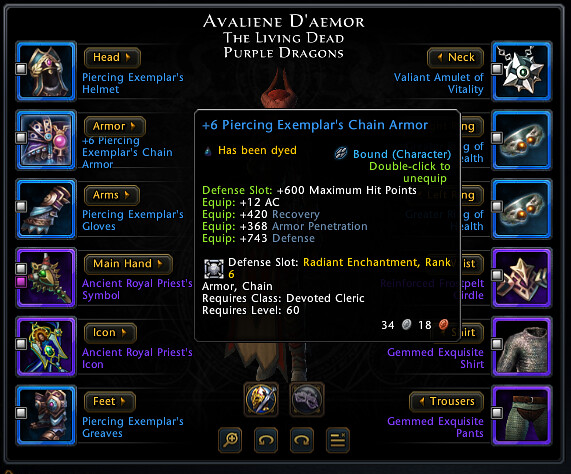This image is a screenshot from an online role-playing video game, resembling the user interface of games like World of Warcraft. The backdrop is predominantly black, with white, purple, and blue text. Centered at the top is the character's name, "Aveline D'Amour, the Living Dead Purple Dragons.” The screen is framed by a series of equal-sized squares in purple and blue on both sides, featuring stylized cartoon depictions of various armor pieces such as headpieces, neck pieces, and trousers, each item's description is color-coded to match its square.

In the middle of the image, a partially obscured 3D cartoon character is visible behind a black box. The box, written in blue text, prominently displays "plus six piercing exemplars chain armor," accompanied by additional specs in green, yellow, blue, and white text. These include attributes like "+600 maximum hit points," "bound to character," "+12 AC," "+420 recovery," "+368 armor penetration," and "+743 defense." Blue and purple colors indicate the rarity of the items. The left side showcases customization slots for head, armor, arms, main hand, icon, and feet, while the right side features slots for neck gear, rings, trousers, and shirts, along with labels and values to further describe each piece of equipment.